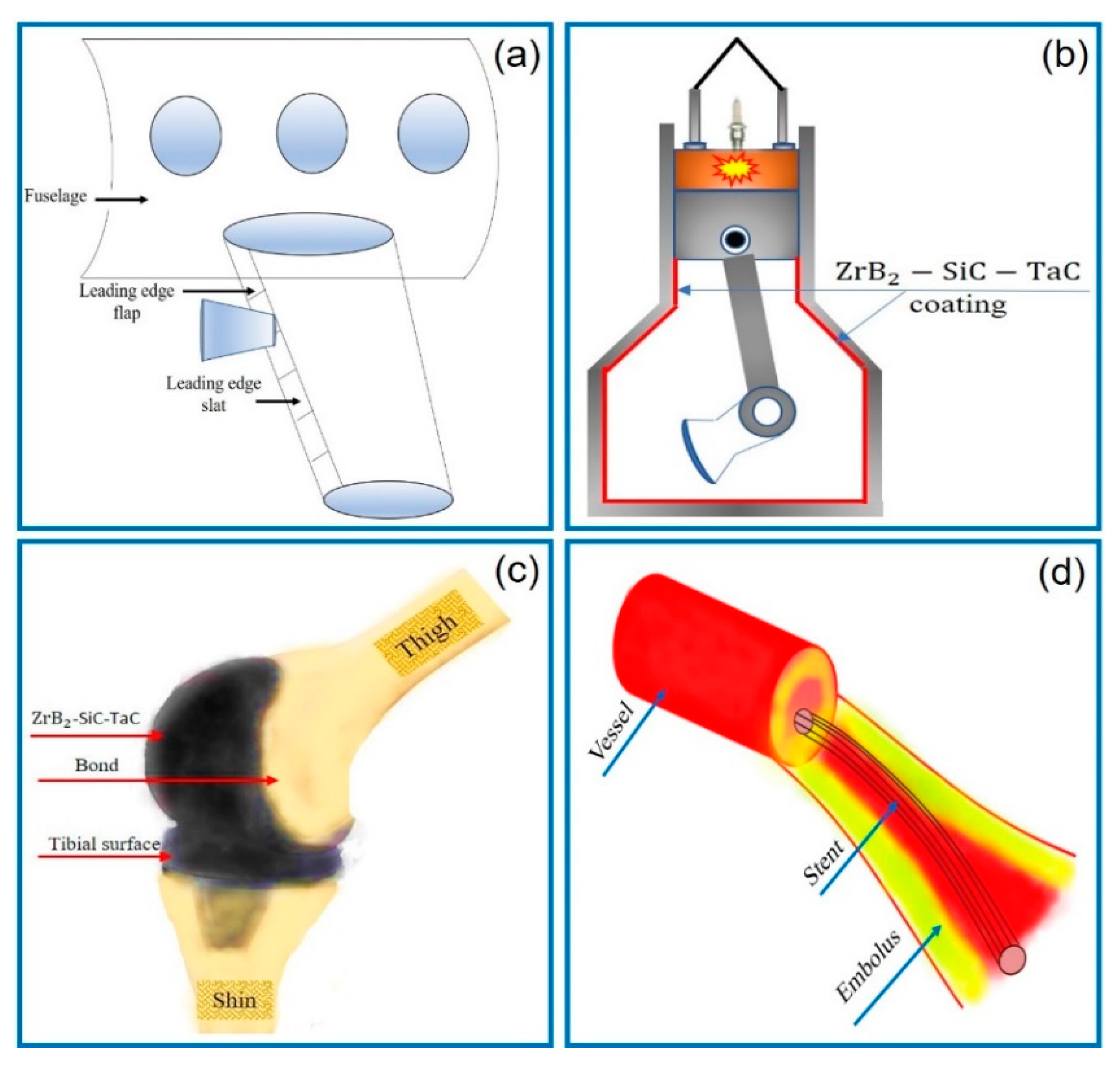This image is a detailed diagram consisting of four quadrant sections labeled A, B, C, and D, each illustrating different parts of various objects and processes. 

Quadrant A, in the upper-left corner, features what appears to be the interior of an airplane. It shows three windows and contains black arrows pointing to terms such as "fuselage," "leading edge flap," and "leading edge slat." There's also a chute or ladder-like structure shown inside the cabin. 

Quadrant B, in the upper-right corner, seems to depict an experiment or mechanical component, labeled with coatings like ZRB2-SIC-TAC. It focuses on a burner and its elements.

Quadrant C, in the lower-left corner, illustrates a medical scenario involving a knee joint. It shows bones labeled "thigh" and "shin" connected, with another reference to the ZRB2-SIC-TAC coating. The terms "bond" and "tibial surface" are used to describe aspects of the bone connection.

Quadrant D, in the lower-right corner, shows part of a blood vessel with a stent inside, identified with terms like "vessel," "stent," and "embolus."

Each section is accompanied by text and arrows pointing to specific parts, making the diagram a complex but informative visual aid for multiple fields, including aeronautics, medical procedures, and experimental sciences.